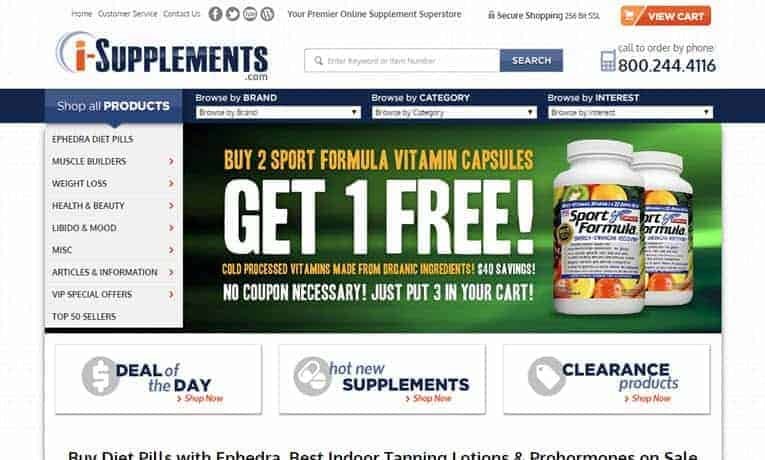In this image, we have a screenshot of the homepage of iSupplement.com. The website name is prominently displayed, with "i" in orange and "supplement.com" in blue, all set against a white background. 

At the top of the page, there are several navigational elements and customer service options, including social media icons for Facebook, Twitter, and email. The site offers customer service help, contact information, and various shipping options. The upper right corner features an orange "View Cart" button. Just below this is a phone icon with the caption "Call to Order by Phone" followed by the number 800-244-4116. To the left of the phone number is a search bar with a blue search button.

Central to the page are browsing options labeled "Browse by Brand," "Browse by Category," and "Browse by Interest," which serve as filters for product searches. 

The focal point of the webpage is an advertisement for a product promotion. It highlights a special offer for "Buy Two Spot Formula Vitamin Capsules, Get One Free." These vitamins are described as cold-processed and made from organic ingredients, offering a $40 savings without the need for a coupon—simply add three to your cart. The promotional text is in yellow and white, placed next to a pill bottle labeled "Spot Formula," adorned with images of fruits.

On the left side, a menu provides quick links to various product categories including "Shop All Products," "Weight Loss," "Health and Beauty," "Misc," "Articles and Information," "VIP Special Offers," and "Top 50 Sellers."

The bottom section of the page features three highlighted offers: "Deal of the Day" on the left, "Host New Supplements" in the center, and "Clearance Products" on the right.

This well-structured layout ensures ease of navigation and draws attention to current promotions and popular product categories.